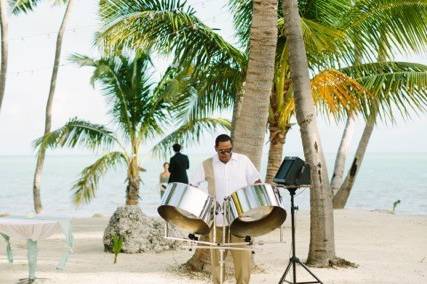The image captures a vibrant scene on a tropical Caribbean beach with a light blue ocean in the background, bordered by an array of palm trees whose heights increase from left to right. The sandy beach is beige and leads up to the clear and somewhat cloudy sky.

At the center of the image stands a black man with short black hair, wearing sunglasses, a white collared t-shirt adorned with a tan stripe on his right shoulder, and matching tan pants. He is deeply engaged in playing a pair of large steel drums that are silver in color and open at the bottom. To his left is a black speaker on a stand providing amplification for his music.

Behind the man, to the left, stands a small table accompanied by a large, irregularly shaped rock about two to three feet high. Further back, slightly hidden among the palm trees, is a man dressed in a formal black suit who appears to be a waiter. Beside him is a woman sitting down, both of whom add to the busy atmosphere of the beach scene. The palm trees behind them vary in size, with smaller ones near the central man and larger ones stretching towards the water's edge, their fronds a mix of green and hints of orange, contributing to the lush, tropical ambiance.

The overall scene is a picturesque blend of music, nature, and human activity against the serene backdrop of a beautiful Caribbean shoreline.